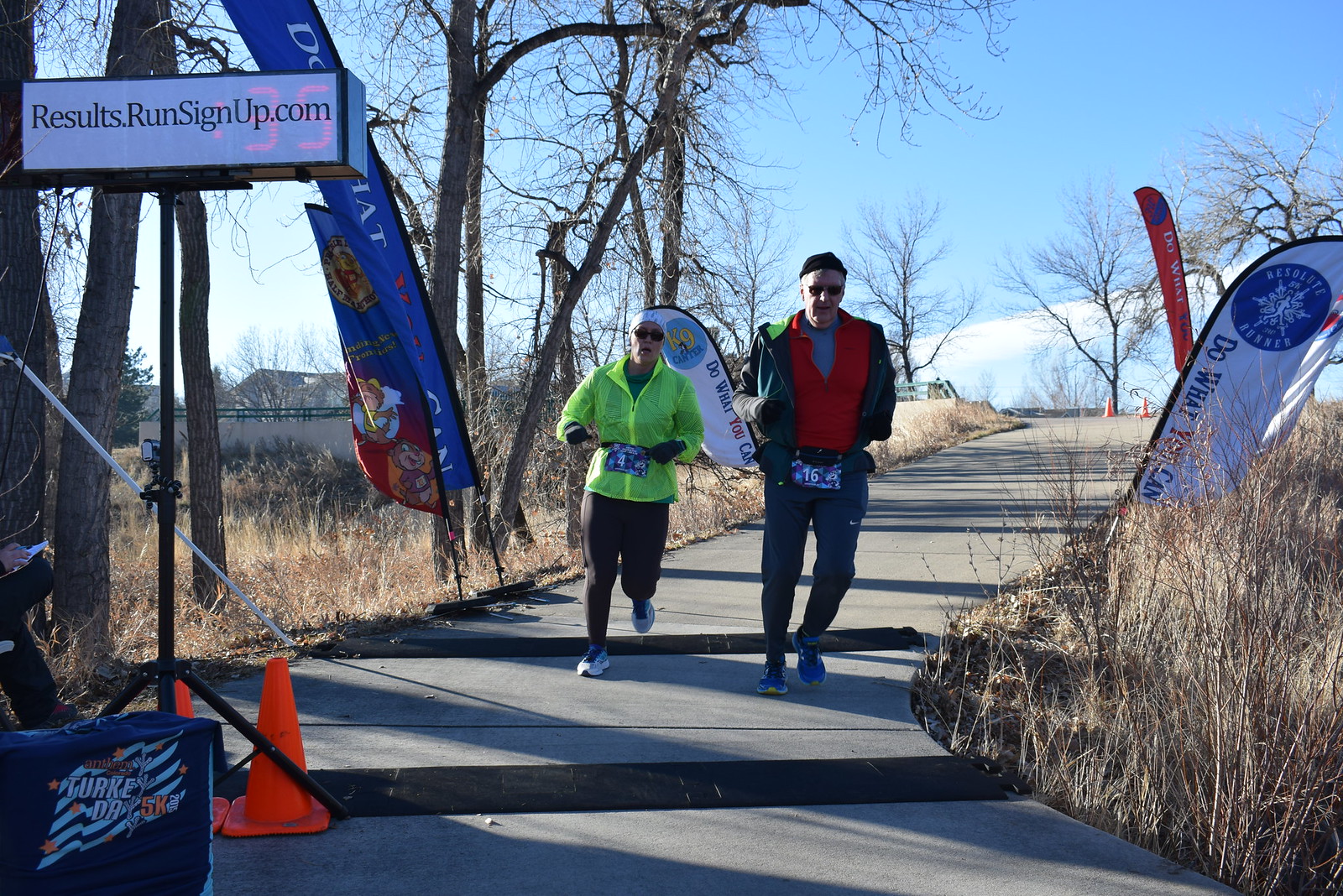In the photograph, an older man and woman are jogging, possibly participating in a marathon or a 5K event given the labels they wear. The woman on the left sports a yellow rain jacket, black pants, white tennis shoes, blue or black gloves, and black sunglasses. She carries a green undershirt beneath her jacket, and her tag reads the number "4" with some indistinguishable white text. The man on the right wears a knit beanie, black sunglasses, a reddish shirt with a greenish coat over it, and a gray turtleneck underneath. He has gray sweatpants and blue and yellow sneakers, with the number "16" on a blue tag at his waist.

The setting includes a gray sidewalk with black sections resembling humps or steps, flanked by brownish grass and leafless trees. Several signs dot the area, including a prominent one in the upper left corner reading "results run signup.com" and another with motivational text: "do what you can," color-coded in blue and red. Orange cones mark the path, suggesting an organized route. In the background, some houses with dark rooftops and an off-white wall are visible under a blue sky with white clouds. The entire scene, marked with signs of cold weather, is likely part of an event subtly branded "Turkey Day 5K" as indicated at the bottom corner of the image.